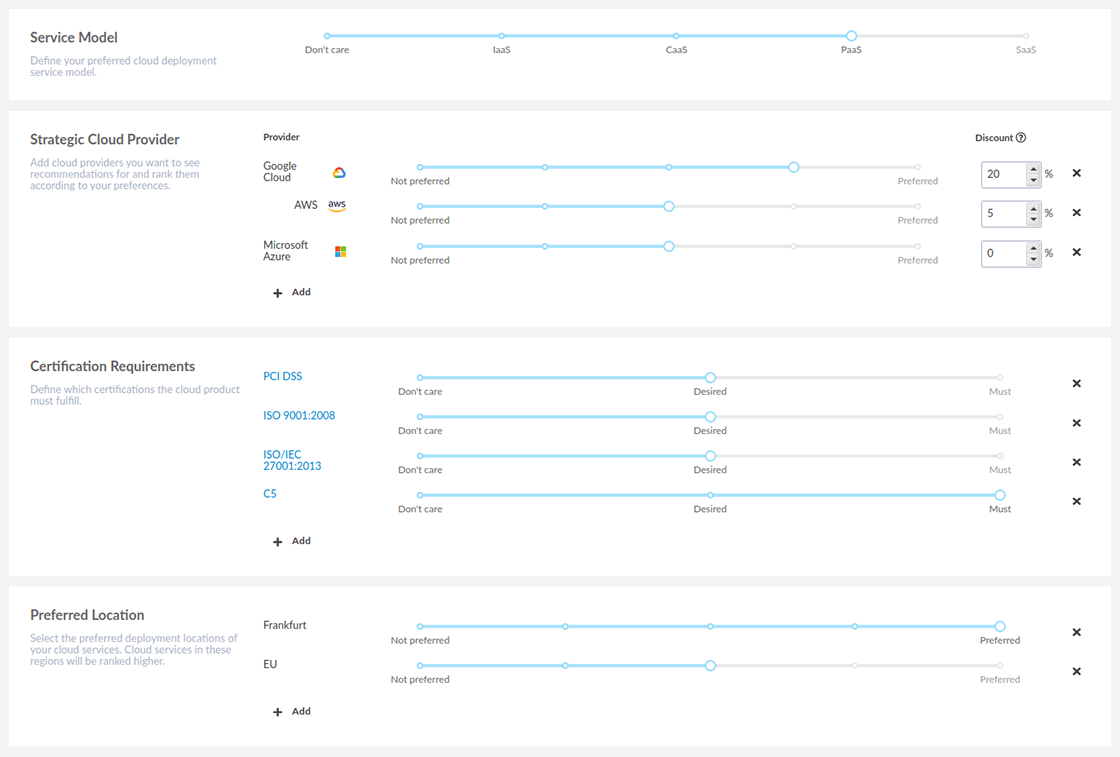In the image, there is a detailed flowchart for selecting and configuring cloud service providers. 

- On the left, in black text, the header reads "Service Model," followed by a long horizontal blue line. Beneath this, the options listed are "Don't Care," "CA," "CMS," and "PAX 5." A dot is positioned directly above "PAX 5."
  
- The next section, titled "Strategic Cloud Provider," instructs users to add cloud providers they wish to see recommendations for and rank them according to their preferences. This section includes the word "Provider" in black, followed by the names of three cloud providers: "Google Cloud," "AWS," and "Microsoft Azure." Three blue lines extend horizontally from this section.

- The third section is labeled "Certification Requirements," which prompts users to define which certifications the cloud product must meet. Listed certifications include "PCI DSS" and "ISO 9001-2008," each accompanied by four horizontal blue lines. One of these lines extends all the way to the right, while the others stop midway.

- The final section is a rectangle labeled "Preferred Location." Users are instructed to select their preferred location for cloud services. The black text lists "Frankfurt," followed by two long horizontal blue lines, one of which spans all the way to the "Preferred" label while the other stops in the center.

This comprehensive graphical layout aids in the detailed configuration and selection of cloud service providers based on service models, strategic preferences, necessary certifications, and geographical location.